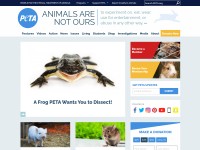This image is a screenshot from a website, featuring a slightly unclear and low-resolution visual quality. The image is notably small, and many of the fonts are blurry and unreadable. At the very top, there's a dark gray header with light gray fonts that are completely illegible due to the blur.

Below this header, the background changes to white, revealing that the website is associated with PETA, the animal rights organization. On the left side, there is a blue circle with "PETA" written inside it in white capital letters, serving as their logo. To the right of the logo, in gray capital letters, the phrase "ANIMALS ARE NOT OURS" is visible. Further to the right, there is some text in a very light gray font that remains unreadable due to the poor image quality. Adjacent to this text, a faint image appears to show a rabbit in a leaping pose.

Continuing down, there's a menu bar featuring multiple items, though their labels are also unreadable. Below this menu, the central part of the screenshot showcases a large photo with a white background. The photo is a close-up of a frog facing the camera, characterized by a dark gray color and an open mouth. Below this image, a headline can be deciphered to some extent, appearing to say, "A Frog PETA Wants You to Dissect."

On the right side of the central image, two smaller photos are present. The top photo possibly depicts the face of a cow, though it is somewhat difficult to ascertain with certainty. The image below it shows what appears to be a guinea pig.

At the bottom of the webpage, there are two additional photos. One is of a small white animal, which might be a rat, while the other shows an animal in green grass, possibly a mouse, guinea pig, or gerbil. Finally, there's another image underneath these two, featuring an animal that could be a mouse. The entire screenshot portrays different animals prominently, reflecting PETA's focus on animal rights and their various campaigns.